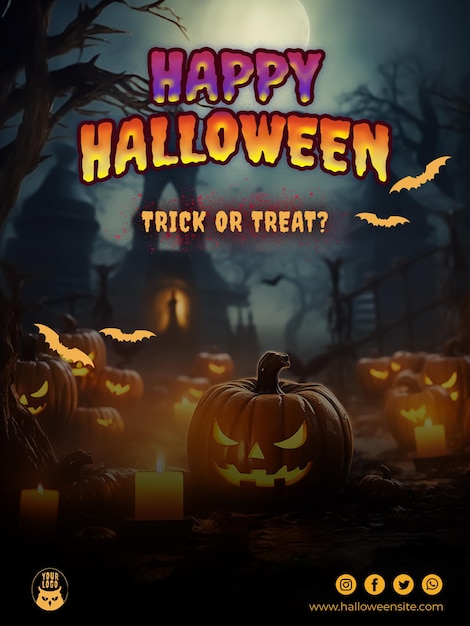A festive Halloween-themed screenshot is filled with various captivating elements. At the top of the image, bold text reads "Happy Halloween," with "Happy" displayed in a striking purple and yellow color scheme and "Halloween" in vibrant orange and yellow hues. Beneath this, the phrase "Trick-or-Treat?" is prominently featured in a similarly vibrant orange-yellow font, punctuated by a question mark.

To the right, several bats in silhouette, depicted in a glowing orange-yellow color, add a spooky touch as they appear to be in mid-flight. A photograph forms the background, featuring an eerie scene at the bottom with numerous jack-o'-lanterns showcasing wicked faces illuminated from within.

In the backdrop, the scene hints at a cemetery with dead, leafless trees and the faint outline of gravestones, enhancing the creepy ambiance. The bottom of the screen displays icons for social media platforms — Instagram, Facebook, Twitter, and one other unidentified icon — along with the website www.halloweenslate.com. Overall, the screenshot seems to be an advertisement for a Halloween event, blending spooky elements with festive flair.